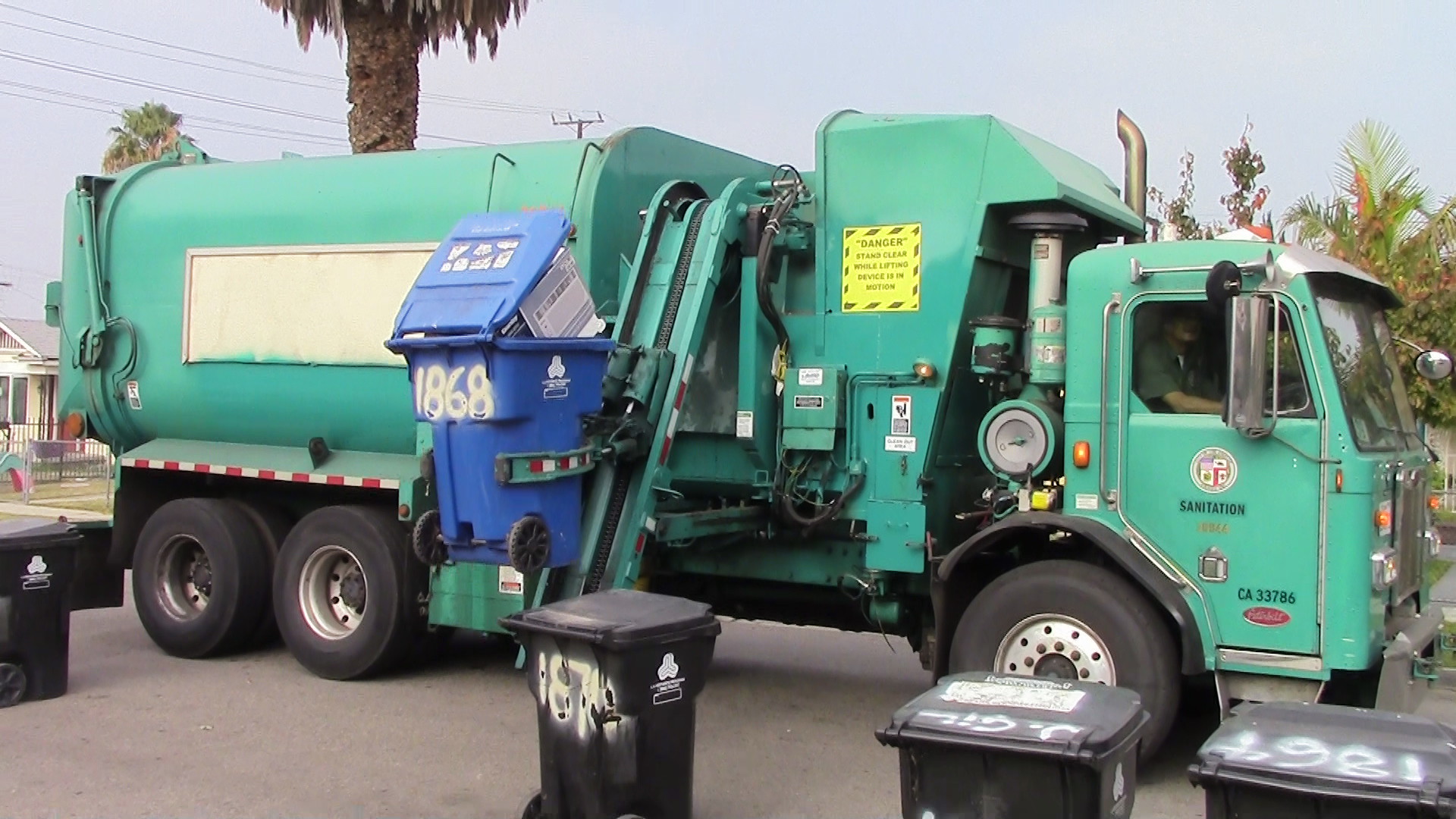The color photograph predominantly features a close-up view of a teal green trash truck, virtually filling the entire frame in landscape orientation. The truck displays the word "sanitation" in black on its front part, which is where the driver would sit. On the right side of the truck, above a red and white emblem and the identification number CA33786, there is a yellow 'danger' sign, although the rest of the text on the sign isn't readable. The truck is equipped with a robotic arm featuring a diagonal conveyor belt at a 45-degree angle, used to lift and empty trash bins. Currently, the arm is lifting a blue bin marked with the numbers '1868' crudely painted in white just below the handles. The bin’s lid is open at a 45-degree angle, revealing contents that include cardboard. The back part of the truck also has a white center, and the truck stands on six large black tires, three on each side. 

The scene is set on a grey tarmac road within a residential neighborhood, evident from houses and a tall palm tree visible in the background. Several additional black trash bins are positioned along the curb in front of the truck, each marked with white spray-painted numbers, possibly addresses.